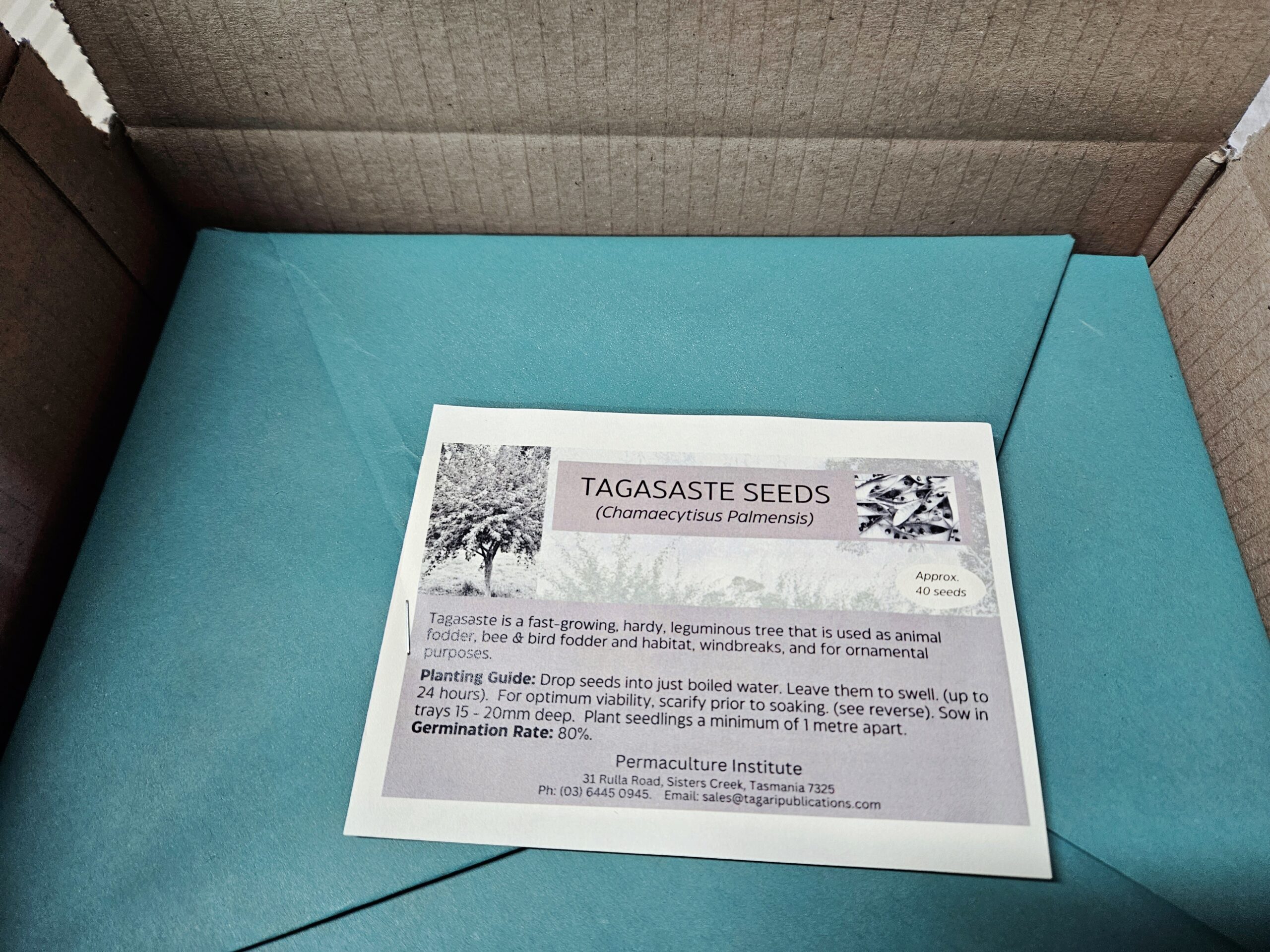The image depicts an open cardboard box with the top flaps undone, revealing a folded, light blue-teal colored paper or fabric on which a printout is placed. The printout, in black, white, and gray, features a detailed description of Tagasaste seeds (Chamaecytisus palmensis). It includes an illustration of a tree and seeds, and text that explains: "Tagasaste is a fast-growing, hardy, leguminous tree used for animal fodder, bee and bird fodder, habitat, windbreaks, and ornamental purposes. Planting guide: Drop seeds into just-boiled water and leave them to swell for up to 24 hours. Scarify prior to soaking for optimum viability. Sow in trays 15-20 millimeters deep, and plant seedlings at least one meter apart. The germination rate is 80%." Additionally, there is a mention of the Permaculture Institute, although further address details are too small to read. It seems the package is intended as a thoughtful gift, carefully prepared and inclusive of comprehensive instructions.